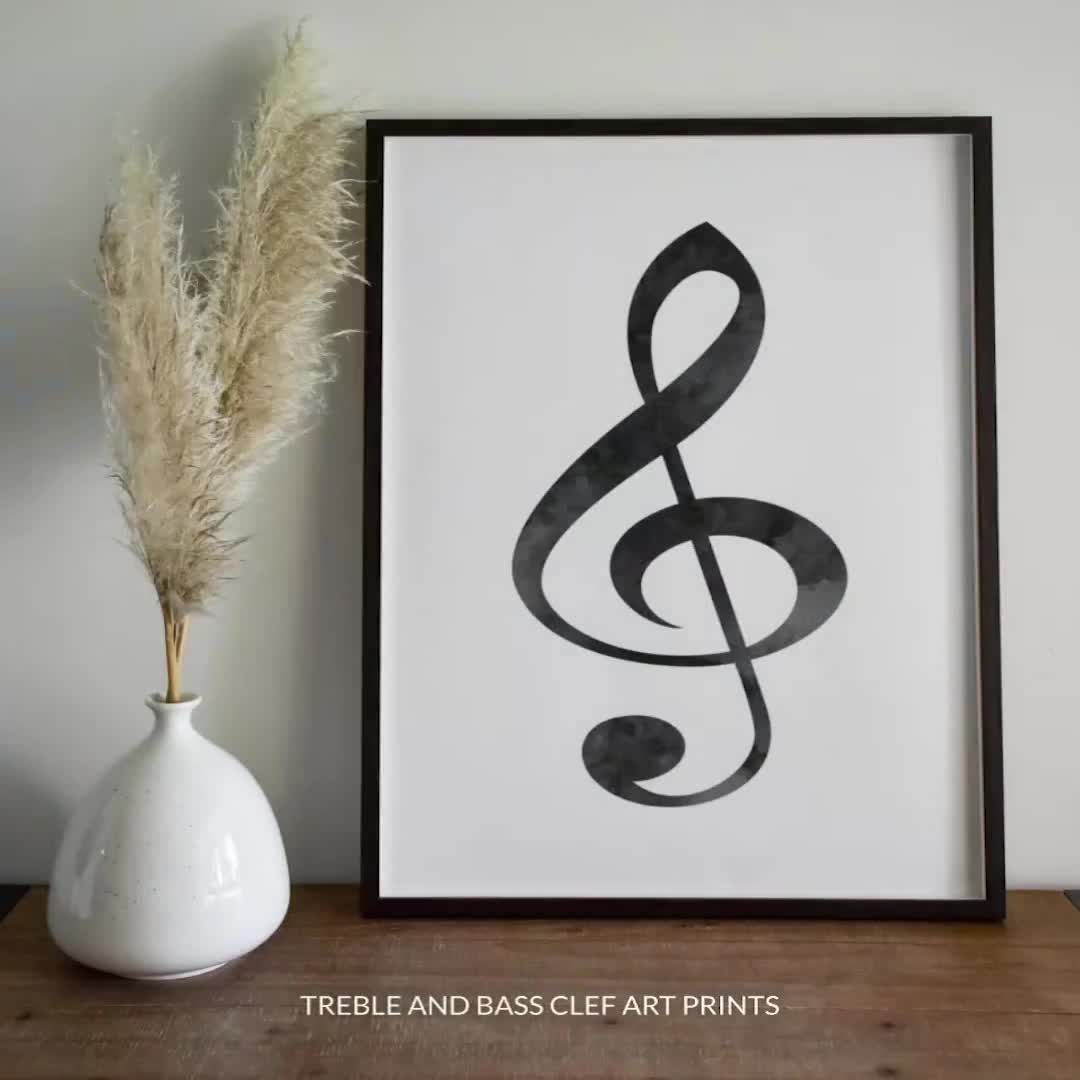This is an indoor product photograph set against a white background, featuring a piece of framed art along with a decorative vase. Centered in the composition is a simple black treble clef printed on a white background, encased in a thin black frame approximately half an inch thick. The frame is leaning against the white wall, supported by a brown table surface. To the left of the art, there is a white, shiny ceramic vase with a small opening at its top from which light brown, feather-like pampas grass extends upwards, reaching towards the top left corner of the image. Subtle shadows cast from the right-hand side add a touch of depth. Near the bottom of the frame, white text reads “TREBLE AND BASS CLEF ART PRINTS,” emphasizing its musical theme. The overall aesthetic is clean, simple, and minimalist, suitable for showcasing in a home setting.